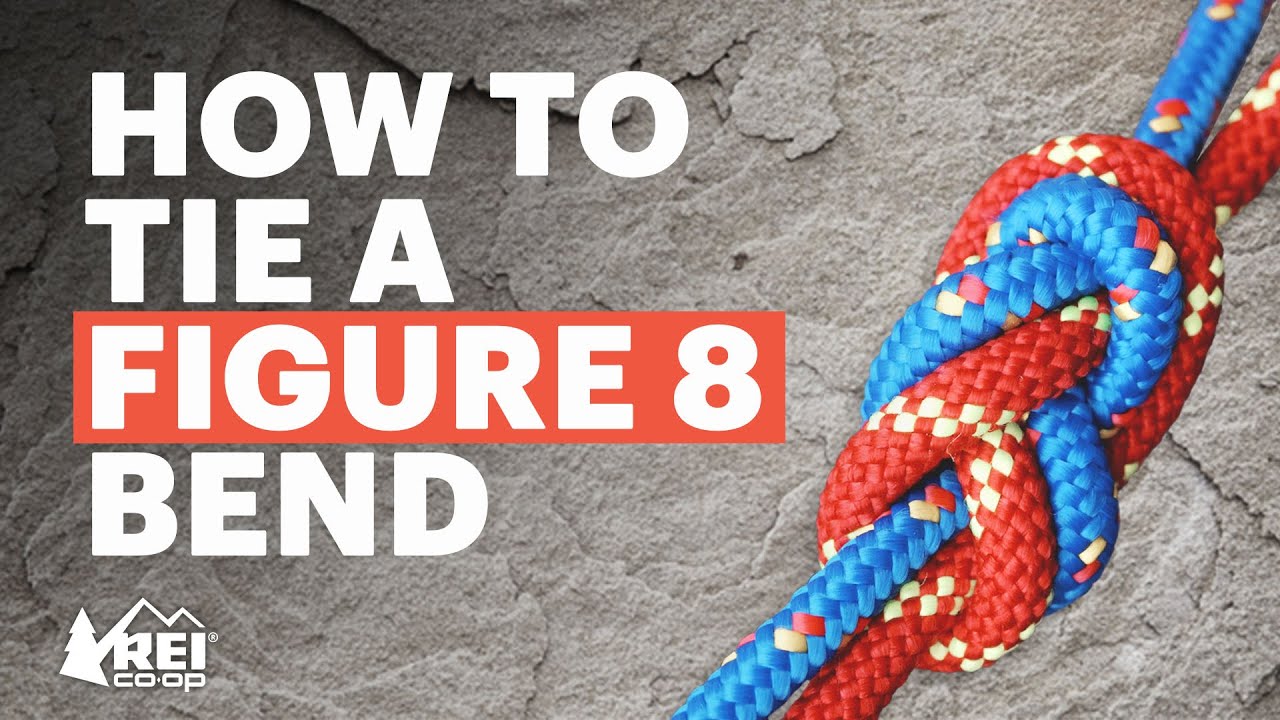The image features an advertisement set against a gray granite rock face, which serves as the textured backdrop transitioning from dark in one corner to light on the other. Dominating the left side of the image, large, bold, capitalized white letters read "HOW TO TIE A," followed by "FIGURE 8 BEND" highlighted with a red background. Below this, the REI Co-op logo is displayed, featuring a white tree silhouette and mountain outline. On the right side, two ropes, one blue and one red, are intricately intertwined in a close-up of a figure 8 bend knot, likely showcasing the ropes’ suitability for rock climbing.